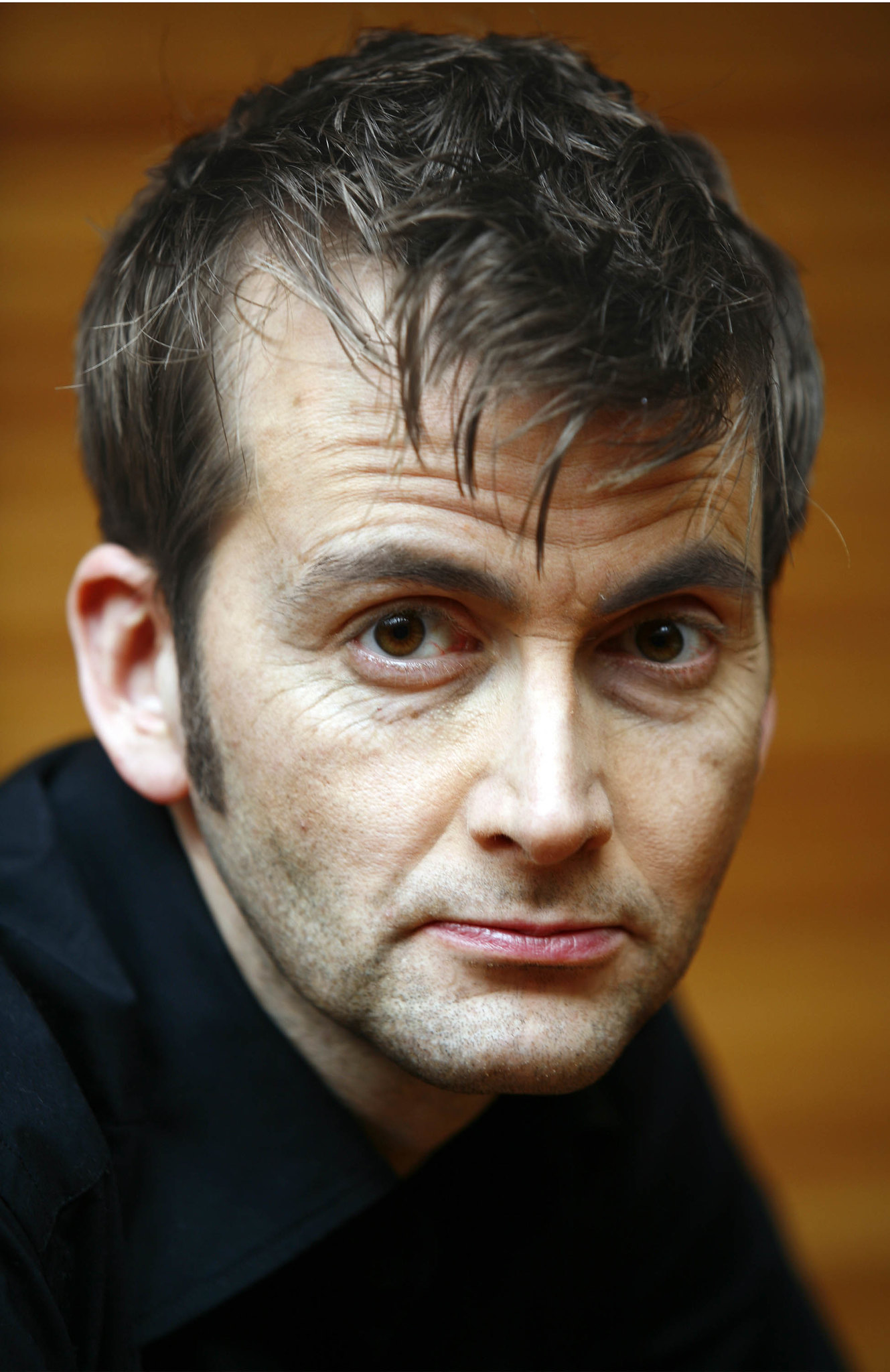The image is a detailed close-up headshot of David Tennant, a white man with fairly pale skin, expressive brown eyes, and a contemplative expression. He has prominent wrinkles on his forehead and around his eyes, giving the impression of deep thought or concern, despite his relatively youthful appearance. His short, somewhat messy brown hair, complete with large sideburns extending to the bottom of his ears, slightly obscures his forehead. His face shows a light stubble, suggesting he hasn't shaved for a day or two, though he maintains a generally clean-cut look. David is dressed in a black dress shirt, which contrasts with the blurred background in varying shades of brown and yellowish light brown, creating a somber and introspective mood in the portrait.